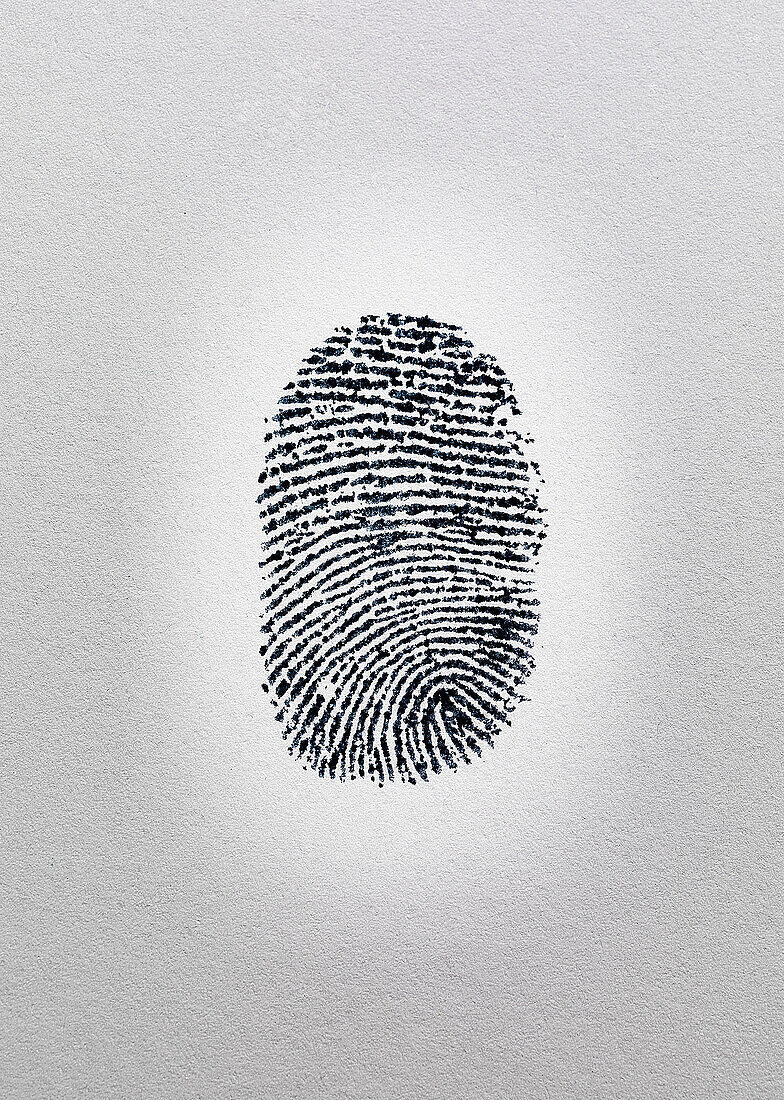The image is a vertically oriented rectangle featuring a close-up of a fingerprint centered against a light gray background that brightens towards the middle. The fingerprint is depicted in black, with intricate patterns that are both unique and varied. The overall shape of the fingerprint is oval, resembling the tip of a thumb. The top part of the fingerprint is dominated by horizontally aligned lines, while the bottom part features lines that are more vertically arched. Some lines extend fully from side to side, while others start at angles and curve upward, creating an intricate series of whorls. Notably, the lower right corner of the fingerprint is characterized by a series of tight whorls, adding to the distinctiveness of the pattern. The surrounding background lightens towards the center, enhancing the focus on the fingerprint.